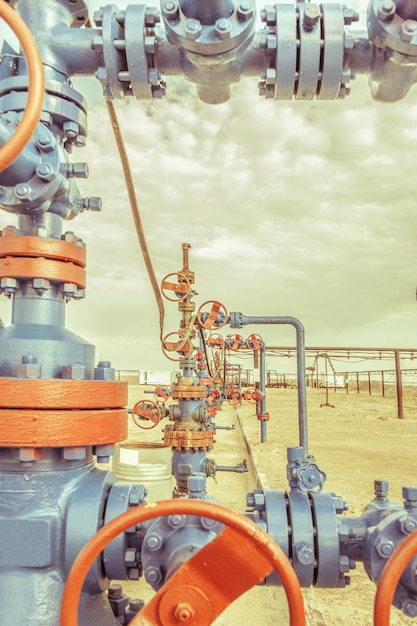The image depicts a complex and intricate network of gray pipes with orange round valves interspersed throughout, creating a striking contrast against a desert backdrop. The overcast, post-apocalyptic sky has a whitish-yellow hue, adding to the eerie yet intriguing atmosphere. Closest to the camera in the lower right corner, two large valves are prominently positioned, while another orange valve is visible in the upper left corner. These pipes primarily run above ground but appear to be connected to mechanisms that lead below the surface, possibly tapping into resources like oil or water. The gray structures with orange trims and the series of interconnected pipes suggest the image could be part of an oil field, water treatment plant, or industrial setup, evoking a sense of both utility and dystopian aesthetics.